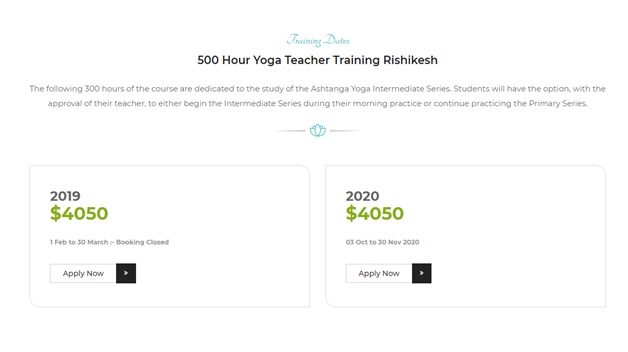A detailed caption for the image could be:

"The image features a segment from the itinerary of a 500-hour yoga teacher training program in Rishikesh. This comprehensive training includes a dedicated 30-hour study of the Ashtanga Yoga and Debate Series. During these sessions, students have the choice, pending approval from their instructor, to either initiate their intermediate series practices or conclude their primary series practices with the Lotus pose. The program offers an in-depth exploration of yoga poses and teaching techniques. Additionally, the image displays textual content alongside graphical elements like bars, potentially depicting progress or scheduling timelines."